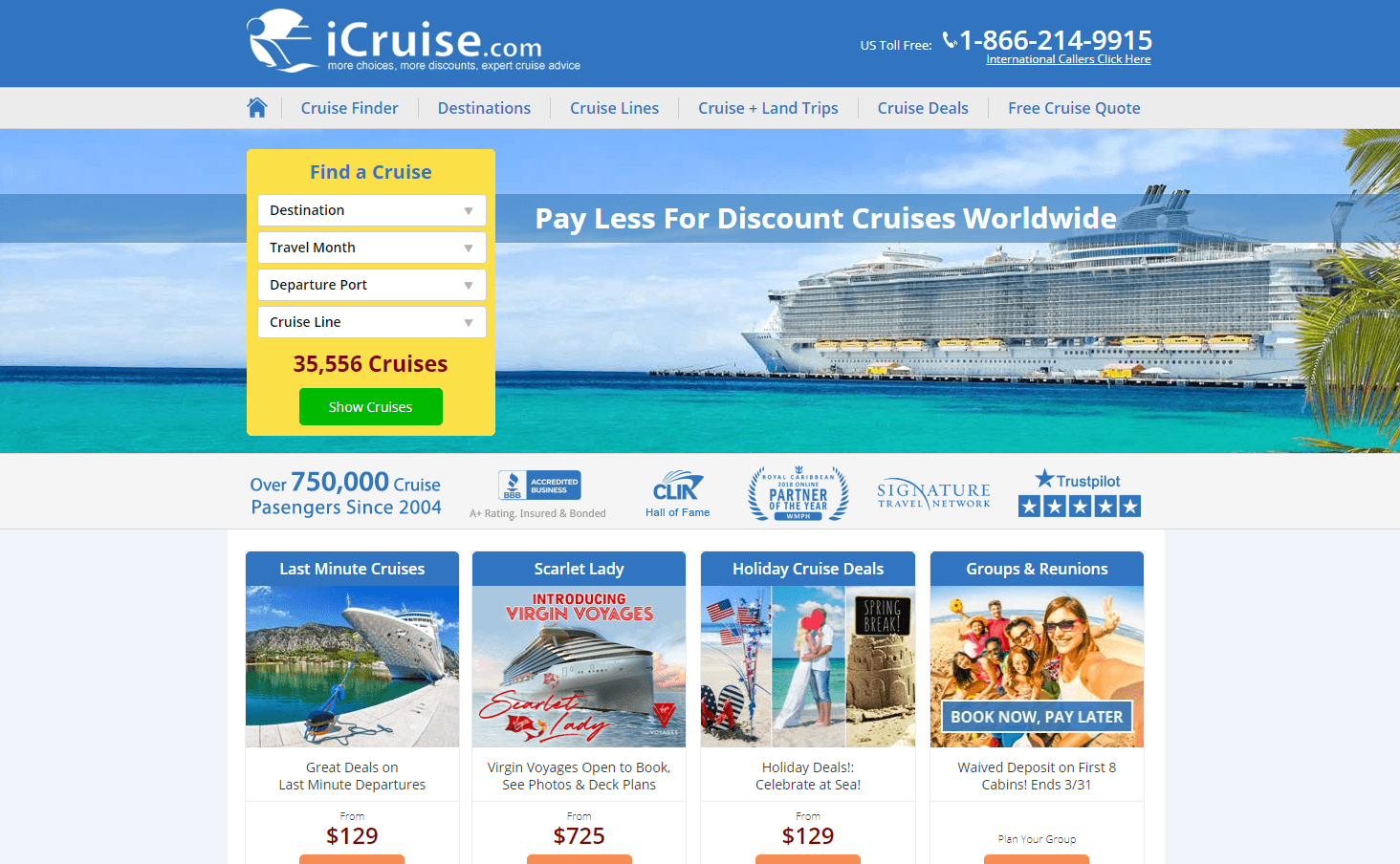The screenshot appears to be from the iCruise.com website. At the top, the background is blue with the website's logo "iCruise.com" prominently displayed in white text alongside a contact phone number. A thick white line separates the logo section from the navigation menu. The menu, displayed in blue text, offers several options: Cruise Finder, Destinations, Cruise Lines, Cruise and Land Trips, Cruise Deals, and Free Cruise Quote.

Below the navigation menu, there is an image featuring a luxurious cruise ship sailing in serene, blue waters. Adjacent to this image, a search box is positioned for users to find their ideal cruise. The fields within the search box include destination, travel month, departure port, and cruise line.

At the lower section of the page, various special offers are highlighted. The offers include Last Minute Cruises starting at $129, a special offer on the Scarlet Lady cruise starting at $725, and Holiday Cruise Deals also from $129. Additionally, there’s a promotion for group bookings and family reunions with the option to "Book Now, Pay Later," featuring a picture of a large group of cheerful people.